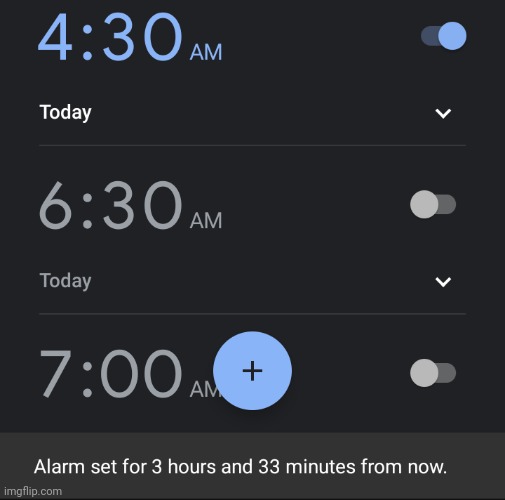The image is a dark-themed, square screenshot from a cellphone displaying the alarm clock settings. Three alarms are visible:

1. **4:30 AM**: This alarm is currently active, indicated by its blue text. On the right side, a blue toggle button confirms its active status. Beneath the time, the word "Today" appears, accompanied by a small arrow pointing downward.
   
2. **6:30 AM**: This alarm is set but not active. It also has the word "Today" below the time, with a grey toggle button and a downward-pointing arrow on the right side.
   
3. **7:00 AM**: This alarm is inactive, evidenced by its grey text and grey toggle button. 

Centered at the bottom of the screen, a large blue plus sign allows the user to add new alarms. Just above this, there's a greyed-out notification with white text, stating, "Alarm set for 3 hours and 33 minutes from now."

In the bottom corner, the watermark "imageflip.com" is visible. The overall screenshot has been formatted into a square shape rather than the typical vertical rectangle of a phone display.